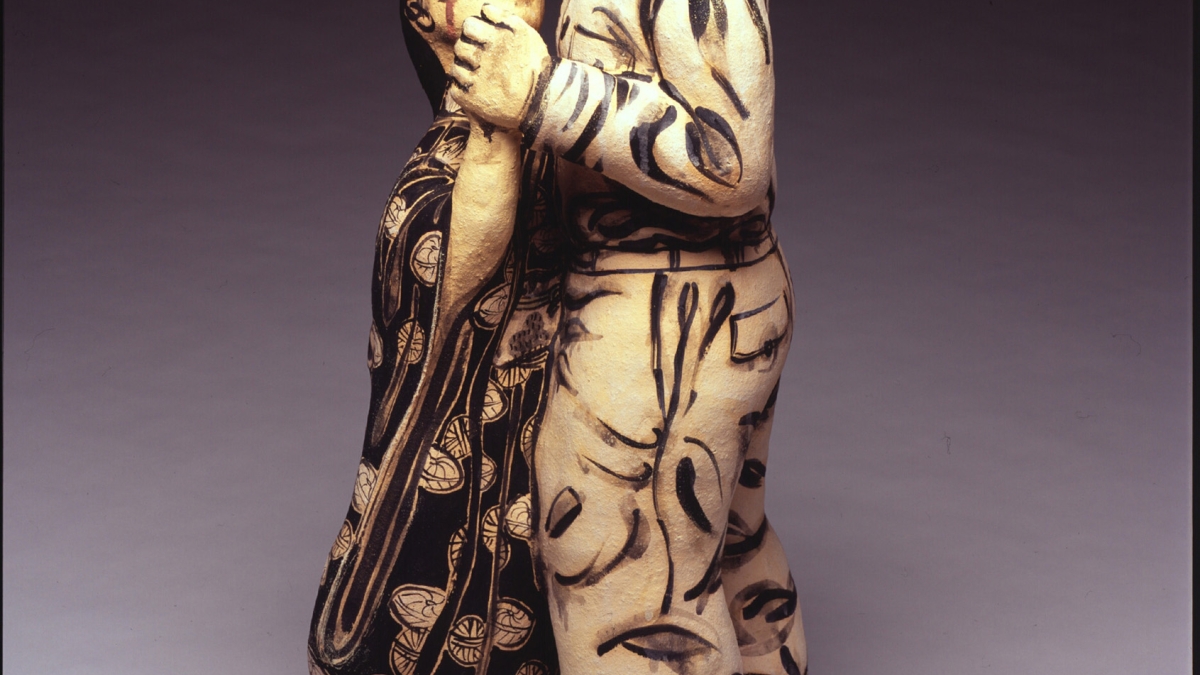The image depicts a detailed close-up of a partial ceramic statue, showcasing two intertwined figures—a man and a woman, seemingly dancing. The statue is carved and painted to evoke an intricate scene; the woman's face is partially visible, adorned with an oversized black dress featuring basket-like designs, possibly floral or fruit motifs. The man's face is entirely out of the frame, and his attire consists of a white ensemble with peculiar black stripes. Both figures are set against a plain, gray background that darkens toward the top, adding contrast to the black-and-white coloration of the artwork. The ceramic texture and the precise depiction of the figures' intertwined arms enhance the sense of movement, making the statue appear almost lifelike despite being only partially visible. Red details highlight the artistic elements, hinting at the depth and craftsmanship of the piece.